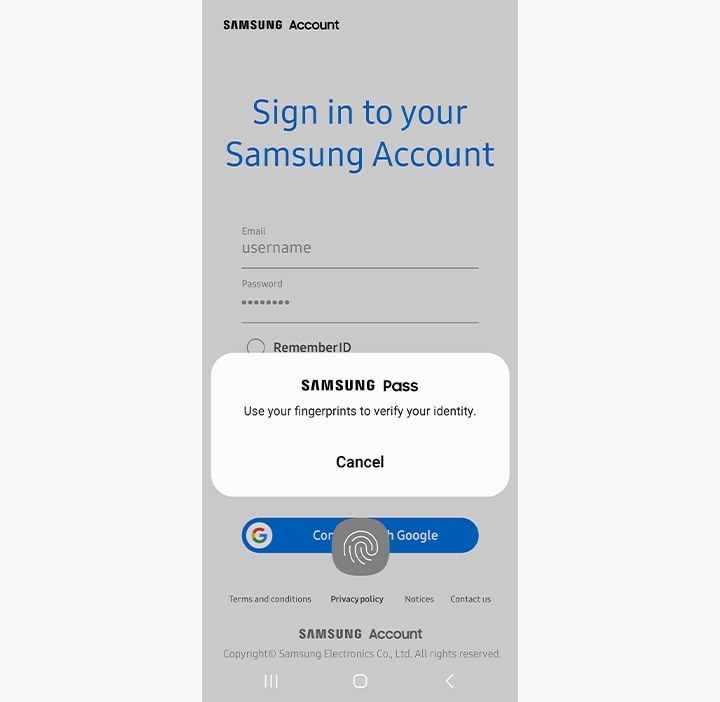The image is a small printout displaying a login screen for a Samsung account. At the top, there's a bold heading that reads "Samsung account." Directly below this, on a gray background, is another heading, "Sign in to your Samsung account." Below this, there are fields labeled "Email," "Username," and "Password," with text indicating that someone's password is entered but hidden from view. 

To the right of the "Remember ID" option is an unselected circular checkbox. Adjacent to this is a highlighted white bar labeled "Samsung Pass," which instructs users to use their fingerprints for identity verification. The options "Cancel" and "Google" appear below, although the latter is partially obscured, showing only the Google logo and the word "Google" in white.

Towards the bottom, still on the gray background, are the links "Terms and Conditions," "Privacy Policy," "Notices," and "Contact Us," listed from left to right. Beneath these links is another line reading "Samsung account," followed by "Copyright Samsung Electronics, LTD, All rights reserved." Finally, at the very bottom, there are three white icons, which look to be clickable.